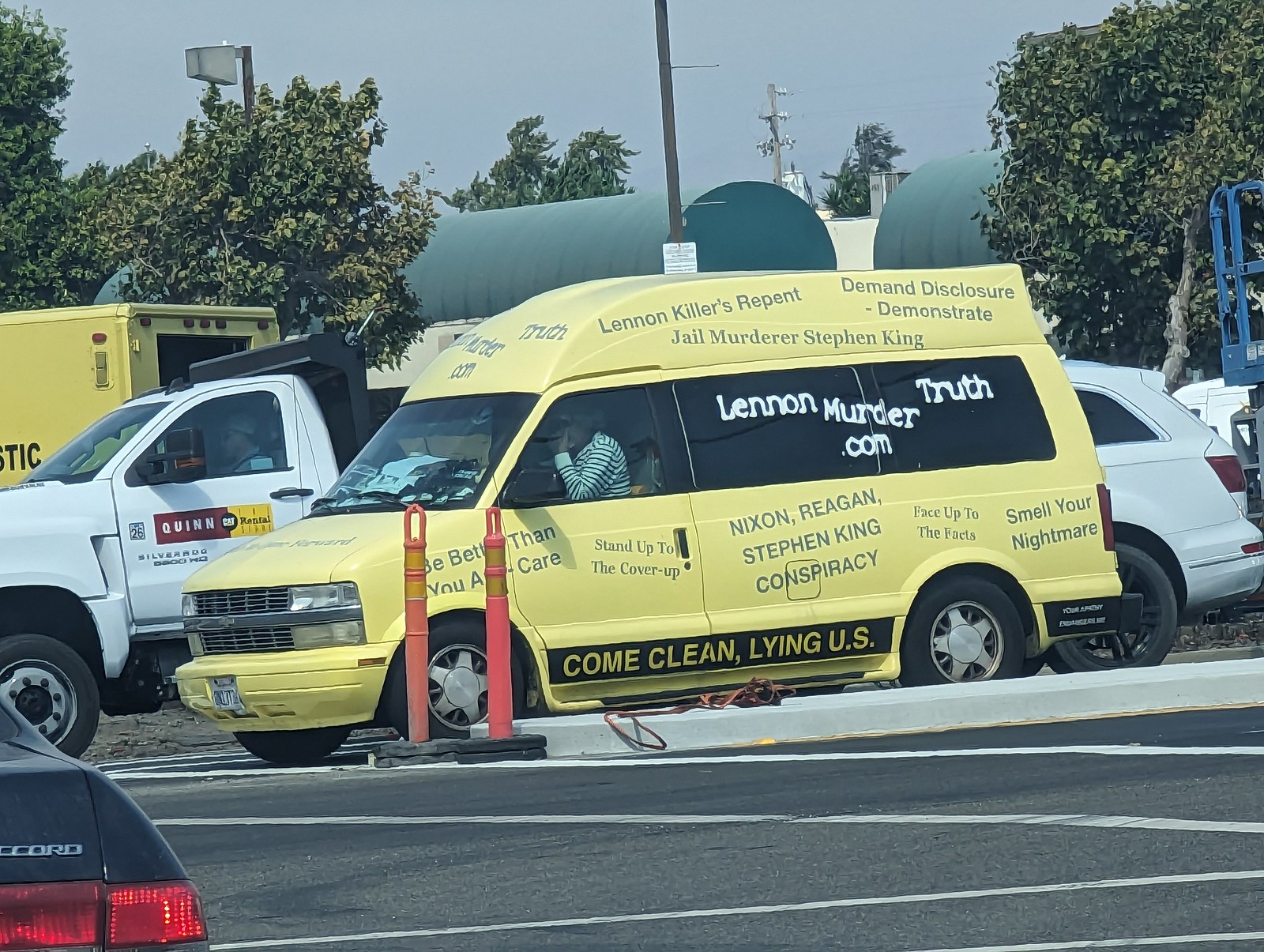This rectangular photograph, shot at an intersection, showcases a striking yellow conversion van laden with conspiracy messages. The focal point, this vivid yellow van, has a higher roof and is adorned with blacked-out, tinted windows. Printed in black and white all over the van are messages such as "Come Clean Lying U.S.," "Lennon Killers Repent Jail Murderer Stephen King Demand Disclosure Demonstrate," "Stand Up To Cover Up," "Nixon Reagan Stephen King Conspiracy," "Face Up To The Facts," and "Smell Your Nightmare." Prominently displayed on the windows is the URL "LennonMurderTruth.com." The van's text is partially obscured by traffic cones and vehicles originating from the intersection. To the left of the van is a white truck with visible "Quinn" branding; further in the background, a couple of larger trucks and trees are visible. A Honda Accord is seen driving through the intersection, against a backdrop of blue sky and trees. An additional white SUV is parked behind the van, emphasizing the everyday nature of this peculiar scene set against black asphalt, complete with parking lines.